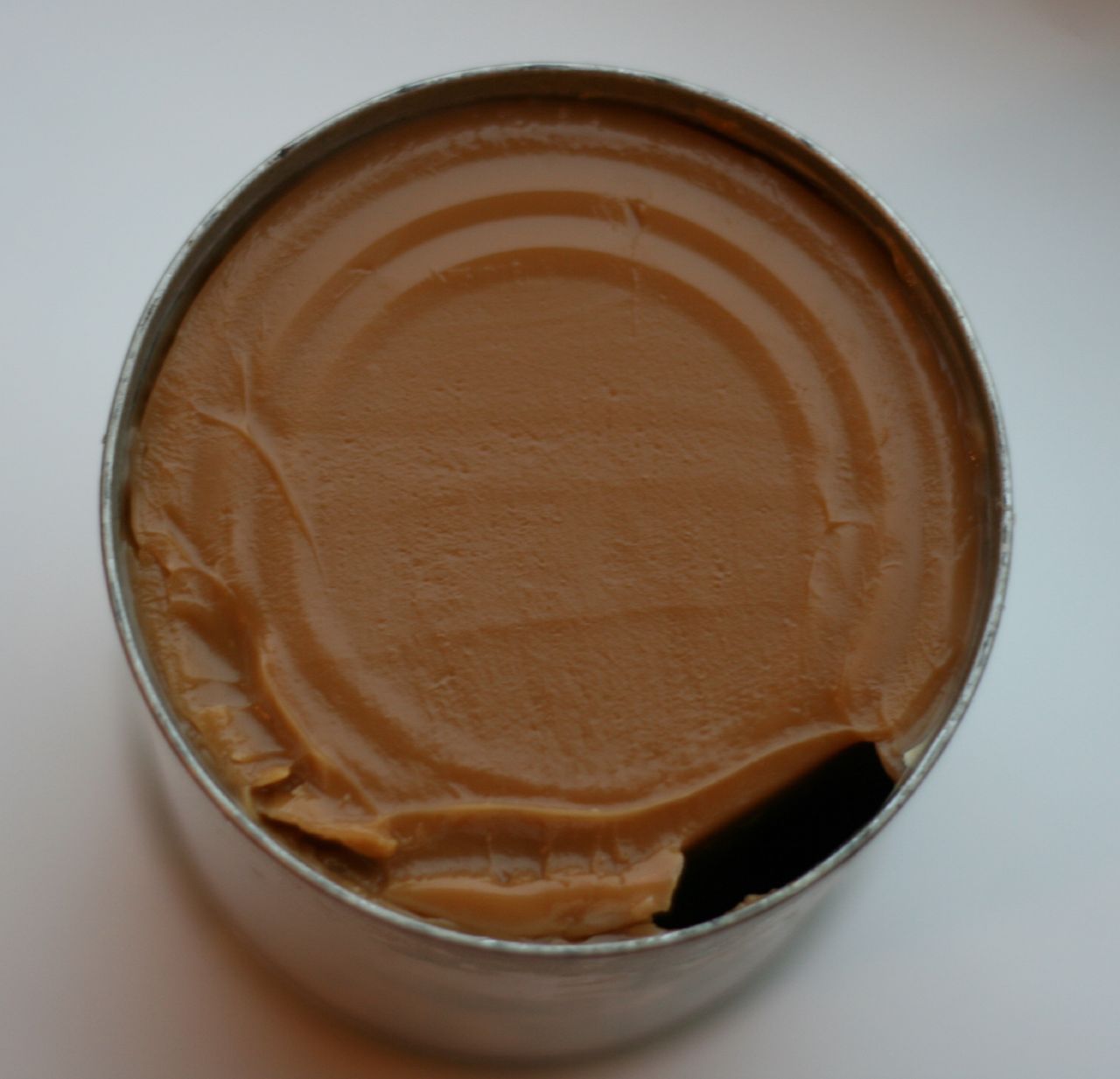A seamlessly opened, standard-sized stainless steel can reveals a dense, thick concentrate within. The substance, which could either be tomato or pumpkin concentrate, displays a varying hue—reddish under certain lights and brownish in others. The smooth removal of the can's lid has left distinct rings imprinted on the surface of the concentrate, suggesting minimal disturbance. A small gap at the bottom indicates a slight shift in the content, allowing a glimpse into the can's depth.